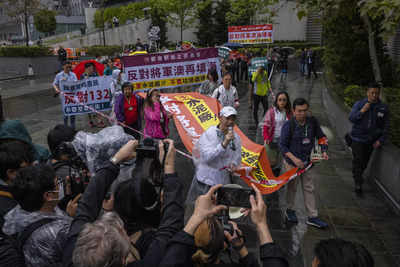The image is a small, horizontal photograph capturing a protest or march, viewed from a slightly elevated angle. A string or line diagonally divides the scene from the upper left to the lower right. On the left side of the line, a group of people, facing slightly to the right and towards the background, are positioned. Many are wearing raincoats and holding up cameras and cell phones, evidently recording the event. Positioned centrally at the bottom, a man dressed in a white shirt and white cap holds a microphone, appearing to be speaking.

On the right side of the line, the protestors hold various large, colorful banners. An orange and yellow banner with black and white writing is noticeable, as well as a banner in the background featuring purple, white, and yellow colors adorned with Asian characters. Another smaller banner with black and red writing is also visible. Beyond the protestors, a sidewalk can be seen with several people walking, and in the background, numerous individuals are visible near a building, adding depth to the scene. The overall backdrop includes trees lining the street, contributing to the urban atmosphere of the setting.